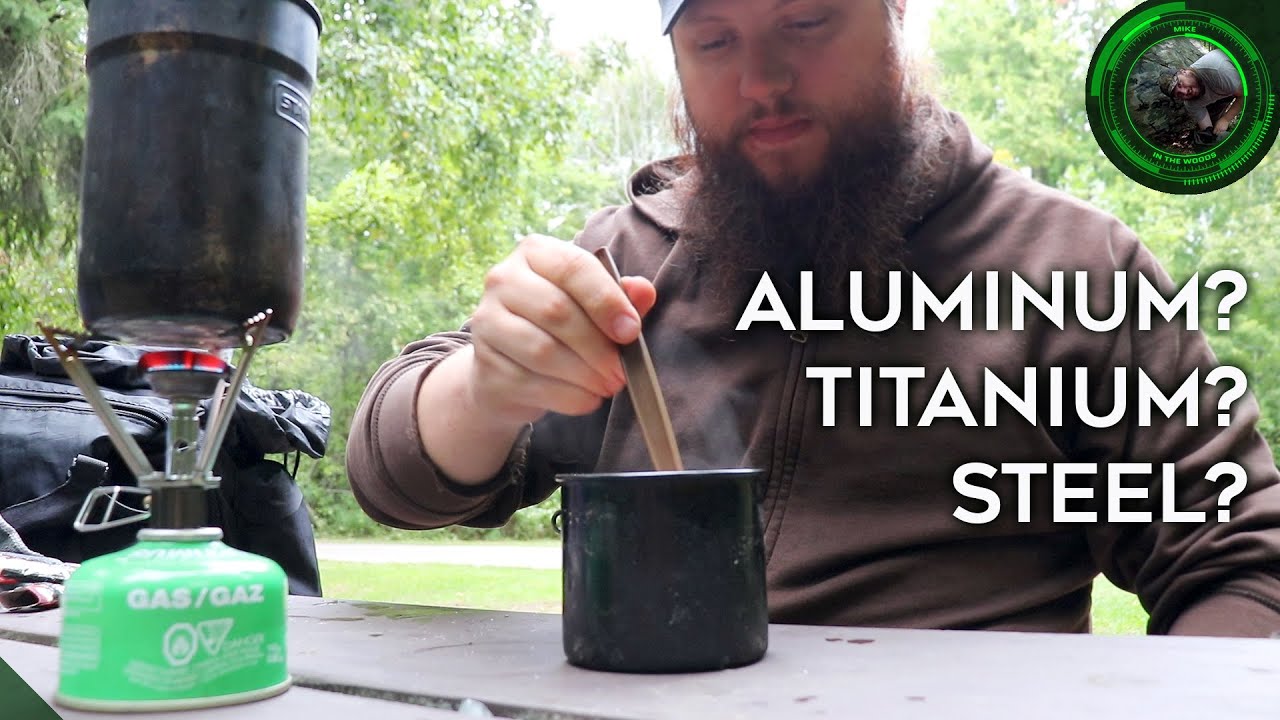The photograph captures a bearded man in a brown hoodie and blue hat, engaging in a material selection experiment outdoors during the daytime. He is stirring a steaming black mug with a spoon, while a green portable gas burner heats another black container on a wooden table beside him. The setting is a lush forest, evident from the green grass and trees in the background. On the right side of the image, white, all-capitals text in a sans-serif font poses three questions: "ALUMINUM? TITANIUM? STEEL?" The top right corner features the website name "Mike in the Woods" alongside a reticle, suggesting this is a YouTube video thumbnail. The scene implies homemade metalworking activity, possibly as part of an educational or experimental demonstration.